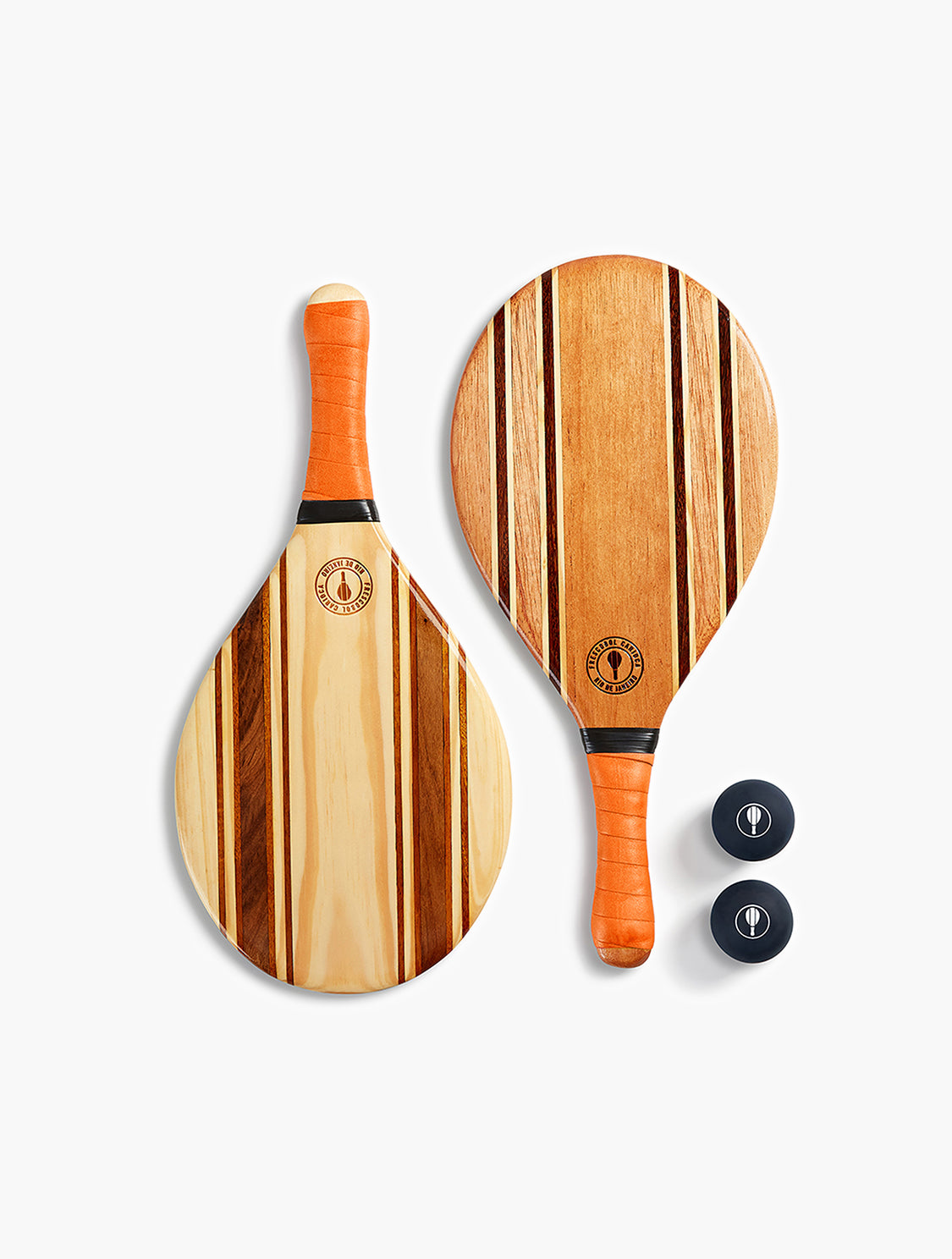The image depicts a beach bat set, consisting of two wooden bats and two dark balls. On the left side are the two bats, each with an orange-hued handle. The bat on the far left has its handle facing upwards and its paddle facing downwards; it features a light brown wood color adorned with darker brown line segments and four thin red stripes. Positioned to the right of it, the second bat is oriented with its handle down and paddle up; it presents a darker wood with intricate patterns. To the right of the bats are two round, dark blue to black balls, each showcasing a small white circle at the center containing a white bat logo. The overall color scheme includes shades of black, orange, light brown, darker brown, beige, white, and touches of red. The setup appears to be a meticulously arranged showcase of ping-pong equipment.